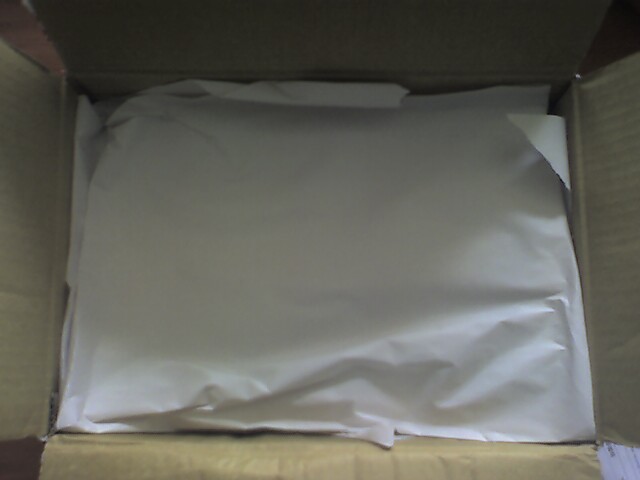The image features an open rectangular cardboard box, with all four flaps unfolded and exposed. Inside the box, there is white construction or wrapping paper that is meticulously folded yet somewhat crinkled and bunched up in areas. The paper seems to be concealing an unidentified item within the box. The surroundings suggest an indoor setting, as the lighting is dim with notable shadowing and a hint of backlighting. The close-up nature of the photo highlights the mystery of the contents obscured by the white paper.